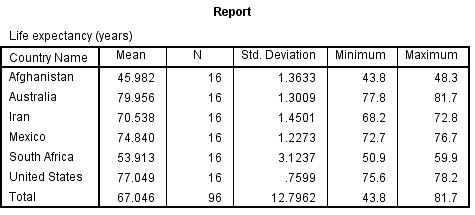The image showcases a detailed life expectancy report against a white background with black text. At the top, the title "Report" is clearly printed in bold. Directly below, it states "Life Expectancy (Years)" above a data table. The table includes columns labeled: "Country Name," "Mean," "N," "Standard Deviation," "Minimum," and "Maximum."

The countries listed are Afghanistan, Australia, Iran, Mexico, South Africa, and the United States, each with respective life expectancy statistics:

- **Afghanistan**: Mean of 45.982 years, N of 16, standard deviation of 1.3633, minimum of 43.8, and maximum of 48.3.
- **Australia**: Mean of 79.956 years, N of 16, standard deviation of 1.3009, minimum of 77.6, and maximum of 81.7.
- **Iran**: Mean of 70.538 years, N of 16, standard deviation of 1.4501, minimum of 68.2, and maximum of 72.8.
- **Mexico**: Mean of 74.840 years, N of 16, standard deviation of 1.2273, minimum of 72.7, and maximum of 76.7.
- **South Africa**: Mean of 53.913 years, N of 16, standard deviation of 3.1237, minimum of 50.9, and maximum of 59.9.
- **United States**: Mean of 77.049 years, N of 16, standard deviation of 0.7599, minimum of 75.6, and maximum of 78.2.

The final row, labeled "Total," aggregates the data with an overall mean life expectancy of 67.046 years for an N of 96, a standard deviation of 12.7962, a minimum of 43.8, and a maximum of 81.7. This table succinctly organizes the life expectancies by country, providing a comprehensive view of statistical measures such as mean, standard deviation, and ranges for the minimum and maximum values.